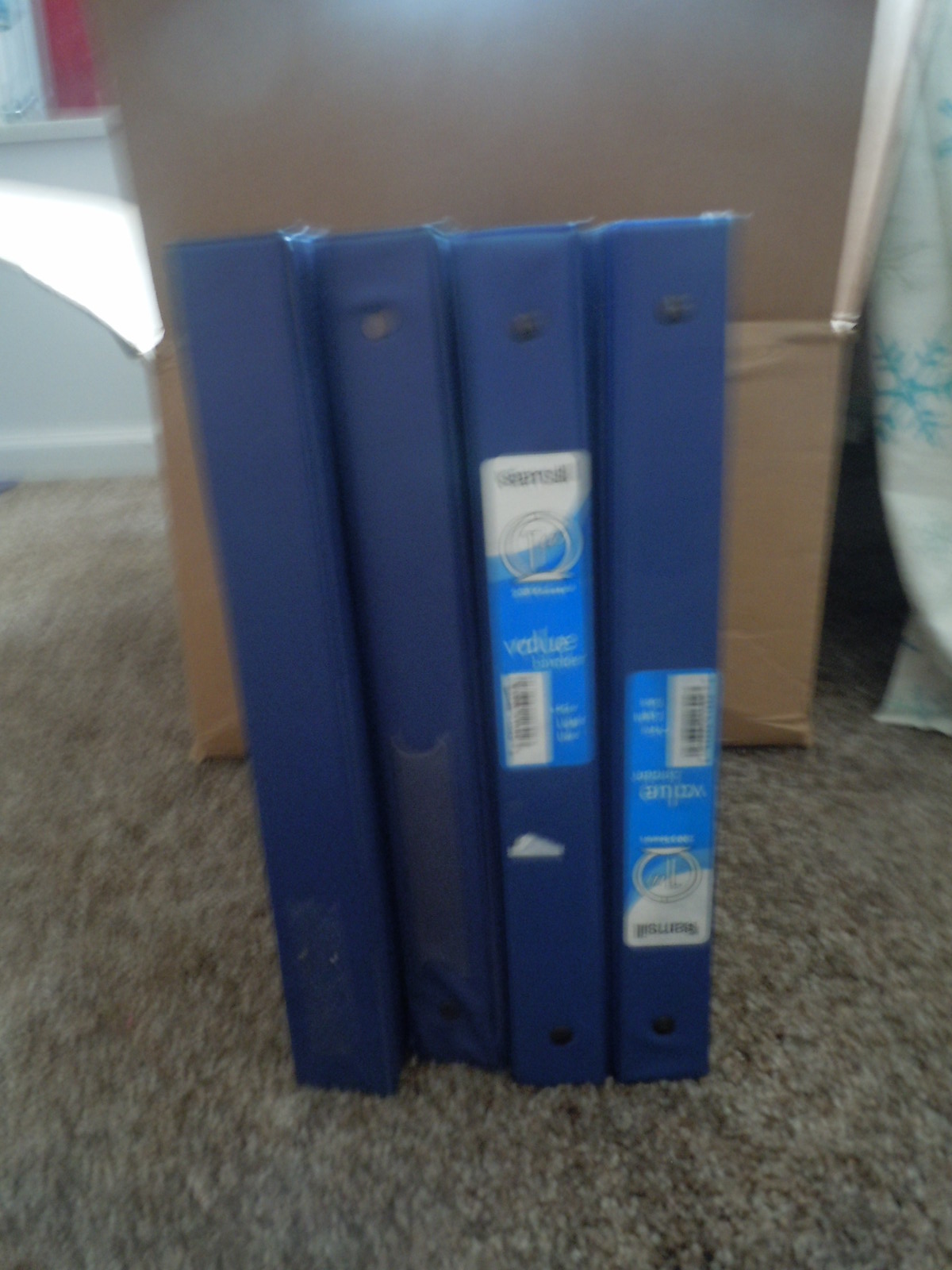This color photograph, taken inside a home, is quite out-of-focus. The image shows four medium blue-colored three-ring binders standing upright on a grayish-brown, mottled carpet. The binders are positioned in front of what are likely two stacked brown cardboard boxes, leaning slightly against them. Behind the boxes, at the bottom of a white wall, sunlight filters in through a window, casting a reflection onto the wall.

The binders are arranged in a line, with their spines facing outward. The first two binders are plain blue without any labels, featuring metallic rivets at both the top and bottom. The third binder also shows rivets and includes a plastic sleeve on its spine, possibly meant for a label. The fourth binder has remnants of a sticky area where a sticker might have once been, but it is devoid of rivets or a plastic sleeve.

In the upper right corner, a piece of fabric with a blue snowflake design can be partially seen, adding a subtle touch of color to the mostly muted background. The photograph captures the everyday clutter of a lived-in space, despite its blurriness.